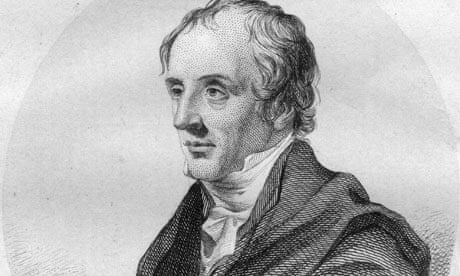This black-and-white illustration appears to be a lithograph or ink sketch intended for reproduction in a magazine or poster. The image depicts a semi-balding white man with longer, slightly wavy hair that falls past his neck. He is shown from the chest up and is oriented in a landscape format, enclosed in a grayish circle. The man is dressed in 18th or 19th century fashion, featuring a flowing, dark coat that resembles a robe, a high-collared white shirt, and a ruffled tie. He is looking in profile from right to left, with a prominent, pointed nose, thin eyebrows, and a neutral expression, gazing slightly away from the viewer. The background is plain, emphasizing the detailed, fine lines and shading characteristic of traditional illustrative techniques like those seen on old currency. There is no text accompanying the image.